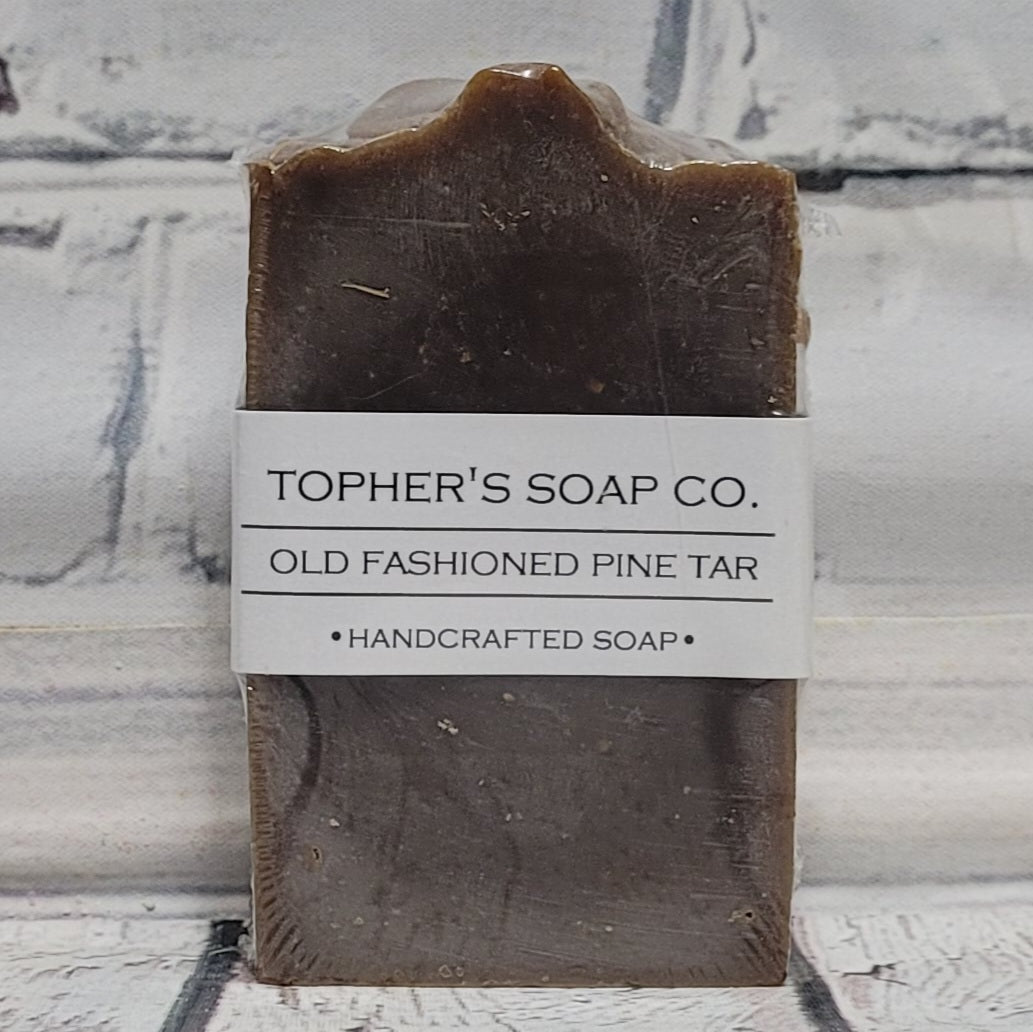In this close-up photograph, a rectangular bar of dark brown soap stands upright, wrapped in clear plastic packaging. The soap bears a thick white label wrapped around its middle, emblazoned with "Topher's Soap Co." in all caps at the top. Below this, a line separates the next line of text which reads "OLD-FASHIONED PINE TAR" in smaller caps, followed by another line. Beneath this line, even smaller caps read "HANDCRAFTED SOAP," flanked by small black dots. The soap rests on a mostly white, textured surface with discernible dark gray grout lines between the tiles. The background is a rough, off-white stone wall with vertical and horizontal striations, creating a slightly rustic, vintage ambiance.